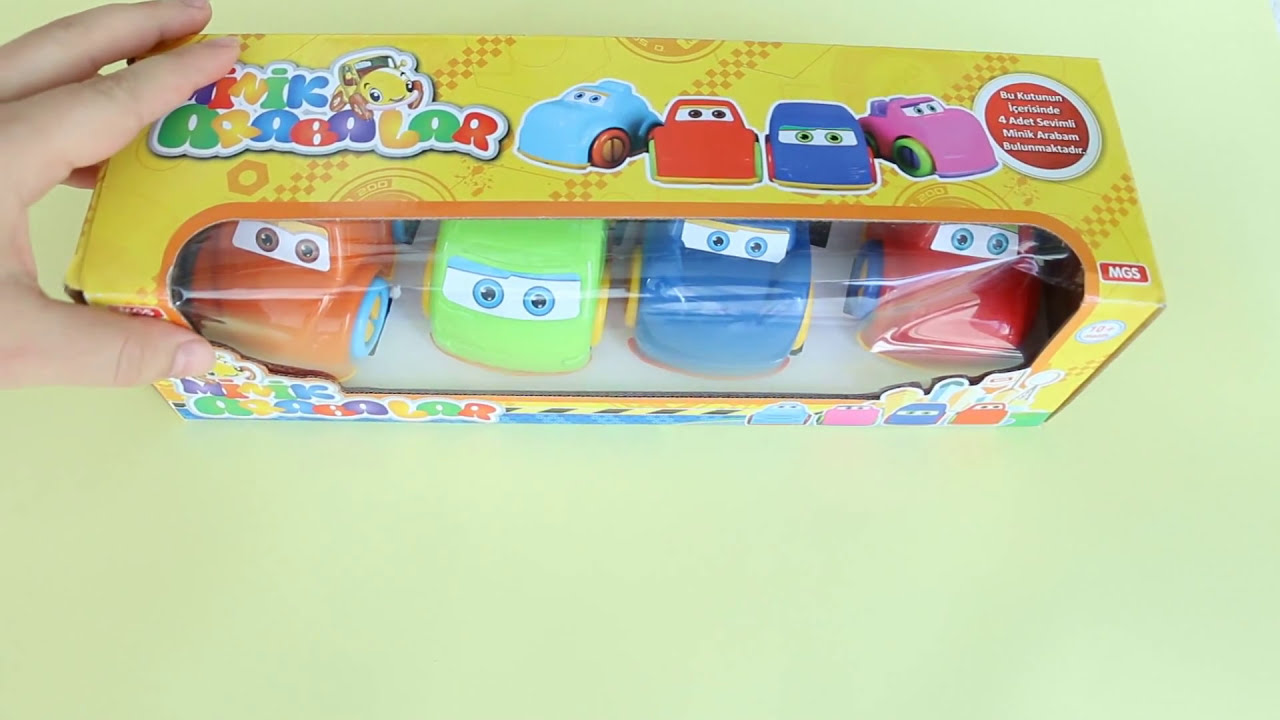The image depicts a white woman's left hand holding and displaying a toy product from an overhead perspective. The product is a yellow rectangular box with colorful graphics and a clear plastic window showcasing a set of four vibrant toy cars inside. The cars are arranged from left to right in the order of orange, green, blue, and red. Each car features a windshield adorned with white stickers depicting blue eyeballs with dark pupils, giving them a playful, anthropomorphic appearance. The box itself has writing in a possibly foreign language, with words that resemble "Inic, Arabellar," and showcases pictures of the toy cars on its top. The background behind the box is a very light green color, making the overall image a horizontal rectangle that is approximately twice as wide as it is tall.